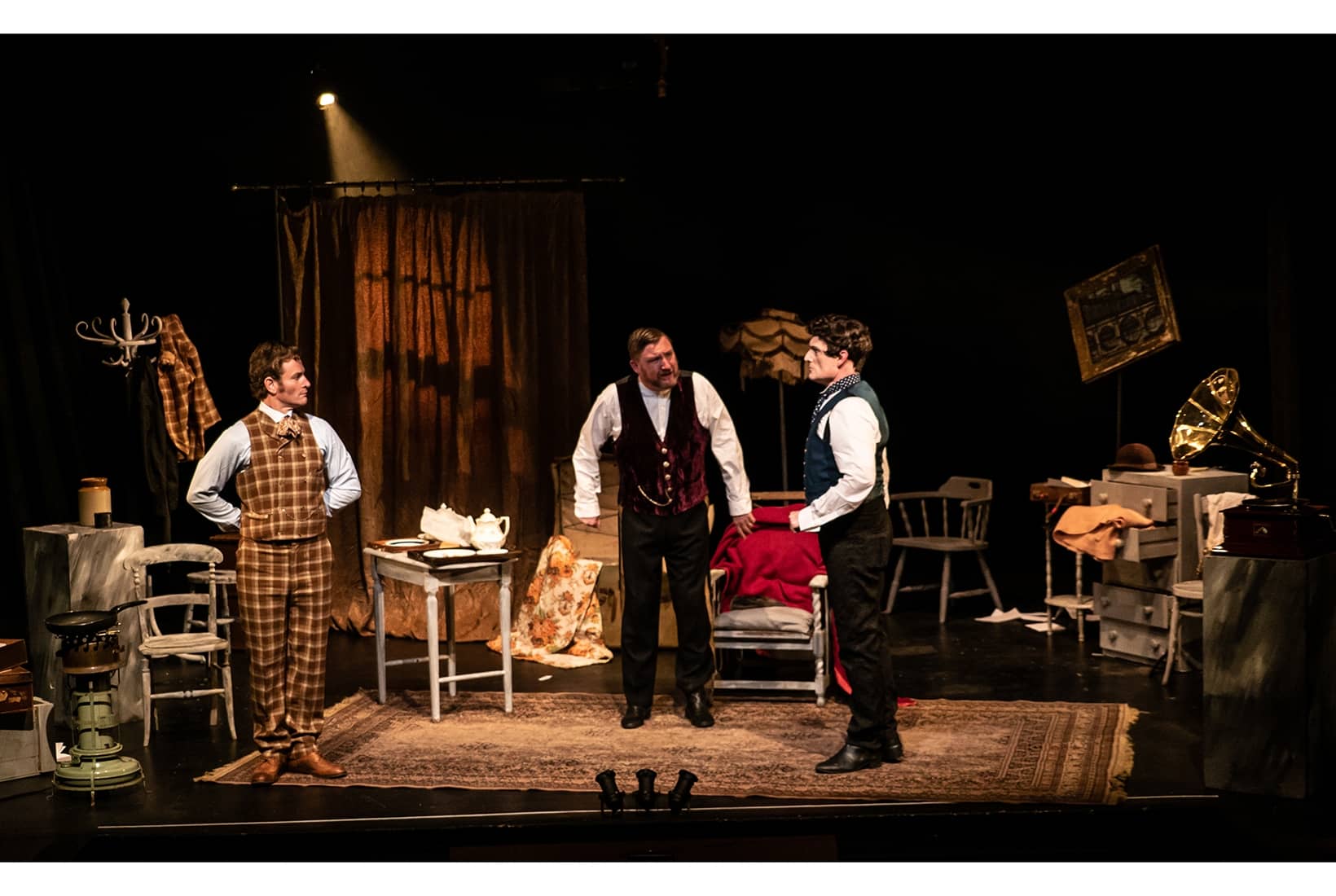In this image, three men are performing on a dimly-lit stage, which is set up to resemble an old-timey living room. Each actor is uniquely dressed in distinct, colorful attire that harkens back to a bygone era. On the left, a man stands in a brown plaid suit, his hands positioned behind his back with elbows jutting out. In the center, another man, appearing agitated, wears a maroon velvet vest paired with dark pants and a white shirt. To their right, facing the maroon-vested man, is a man in a blue vest, white shirt, and dark-colored pants and boots, with a profile that suggests an ongoing conversation or argument. The stage is furnished with a well-worn brown and white rug underfoot, various chairs, a couch, a table, and a scattered assortment of accessories including a gramophone to the far right, enhancing the vintage ambiance. A coat rack with a hanging coat is situated on the left side, and a chest of drawers, with some items partially exposed, is on the right. The background features a floor lamp flanked by dark walls, which adds to the shadowy, intimate effect of the scene.